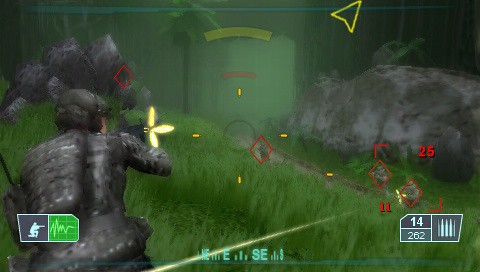This screenshot from an early-version or low-resolution video game captures an action-packed moment in an army-themed shooter. The graphics are simplistic and lack the realism found in modern games, suggesting it might be an older title or one with intentionally retro visuals. In the bottom left corner, a player character is firing a weapon, with ammunition visibly ejecting from the gun. The character is targeting a cluster of small enemies on the right side of the screen, each marked with a red diamond-shaped indicator to highlight them as hostile targets. The overall scene conveys the intensity of the gameplay despite the dated or minimalist graphic style.